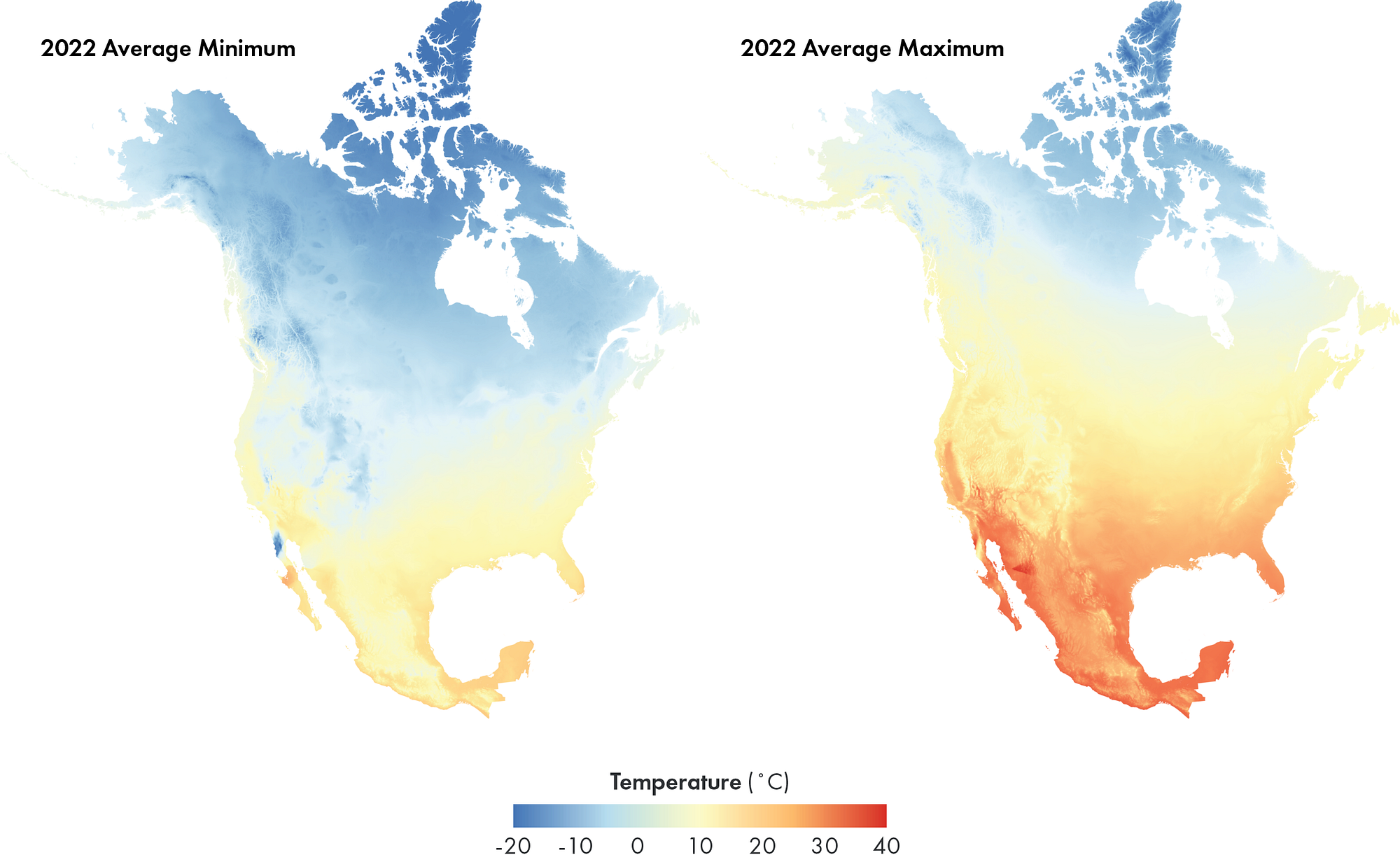The image presents two detailed heatmaps displaying the average minimum and maximum temperatures of North America for the year 2022. On the left, the map illustrates the average minimum temperatures, predominantly shaded in cooler tones with few areas in the warmer orange hues, mainly concentrated in the southern regions. On the right, the map depicts the average maximum temperatures, revealing a more extensive presence of warmer colors, especially vibrant oranges and reds, indicating higher temperatures prevalent from the south of the United States down through Central America. A temperature scale at the bottom of the image ranges from -20°C in blue to 40°C in red, offering a clear visual gradient of temperature intensities.